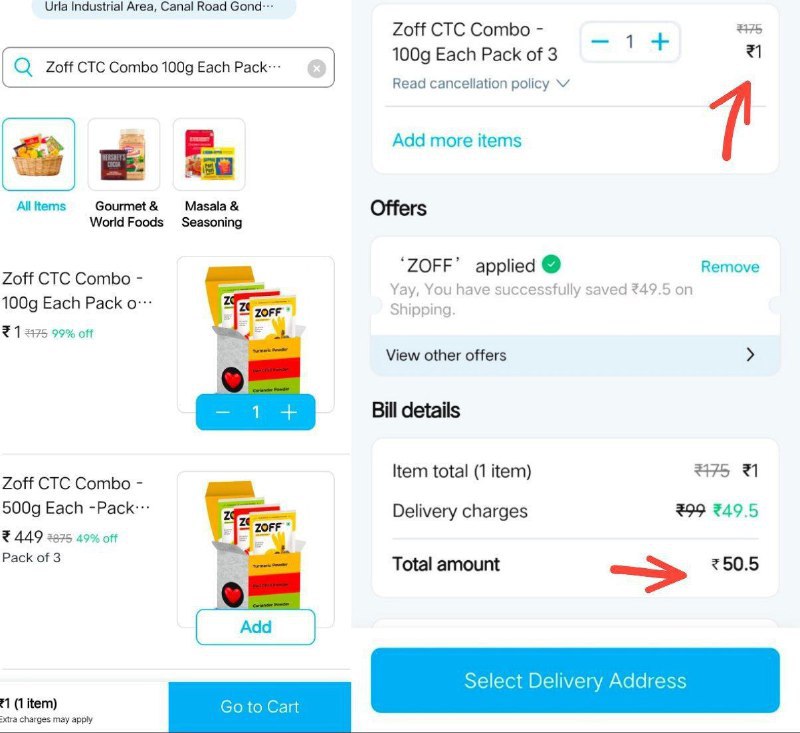This is a screenshot from an unknown website or app displaying a user's shopping page. On the left, the address bar shows the location: Erla Industrial Area, Canal Road, GOND... The search bar indicates the user has searched for "Zoff, Z-O-F-F, CTC Combo, 100G each pack."

Below the search bar, there is a photograph of a wicker basket filled with various bags of food, with the label "All items" selected. Beside the basket image, another photograph showcases a tin of Hershey's cocoa and a jar of an unidentified substance, categorized under "Gourmet and World Foods." Next to this, a third image features a packet and a box of unknown food items, labeled "Masala and Seasoning."

Beneath these images, there is a deal for "Zoff, CTC Combo, 100G each pack," originally priced at 175 rupees, now offered at 1 rupee with a 99% discount. A colorful, illustrated box in red, green, and yellow, filled with unknown packets, is positioned to the right, indicating one item selected.

Further down, a similar photo with the label "Add" appears alongside the "Zoff, CTC Combo, 500G each pack" priced at 449 rupees (originally 875 rupees, with a 49% discount). This deal indicates a "pack of three."

The user is reviewing the cart on the right side of the screen, showing "Zoff, CTC Combo, 100G each pack of three" with the cancellation policy mentioned. One item has been selected at the discounted price of 1 rupee (originally 175 rupees).

Additional notes show a red arrow pointing at the "one rupee offers" with the text "Zoff applied, remove." Celebration text, "Yay, you have successfully saved 49.5 rupees on shipping," and "few other offers" are shown.

The bill details mention:
- Item total: 1 item at 1 rupee
- Delivery charges: originally 99 rupees, now 49.5 rupees
- Total amount: 50.5 rupees

Another red arrow points at the total amount. Lastly, the section "select delivery address" is displayed at the bottom of the screenshot.